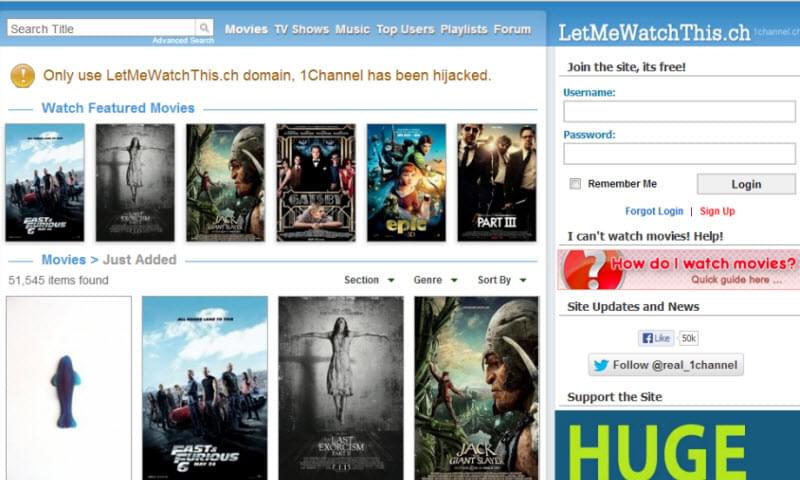The image showcases a user interface with a blue border at the top. On the left side, there is a search bar with the placeholder text "Search Title," accompanied by a magnifying glass icon. Next to the search bar, a menu offers options categorized as "Movies," "TV Shows," "Music," "Top Users," "Playlist," and "Forum."

On the right side, the text "LetMeWatchThis.ch" is displayed prominently. Below this, there is a section encouraging users to join the site for free. It prompts for a username and has a corresponding text box. Following this is another text box for the password, with a "Remember Me" checkbox available for selection. Below these fields is a gray "Login" button, and adjacent to this is a blue hyperlink labeled "Forgot Login." A red link stating "Sign Up" is also present.

Further down, there is a help section with links saying "I can't watch movies, Help," "How do I watch movies," and "Quick Guide here." Additionally, there is a section for "Site Updates and News."

Social media buttons are also featured, including a Facebook "Like" button showing "30k" likes, and a Twitter button inviting users to follow "@real_onechannel."

Finally, there is a banner urging users to support the site, displayed within a blue box that has the word "Huge" written in large yellow letters.